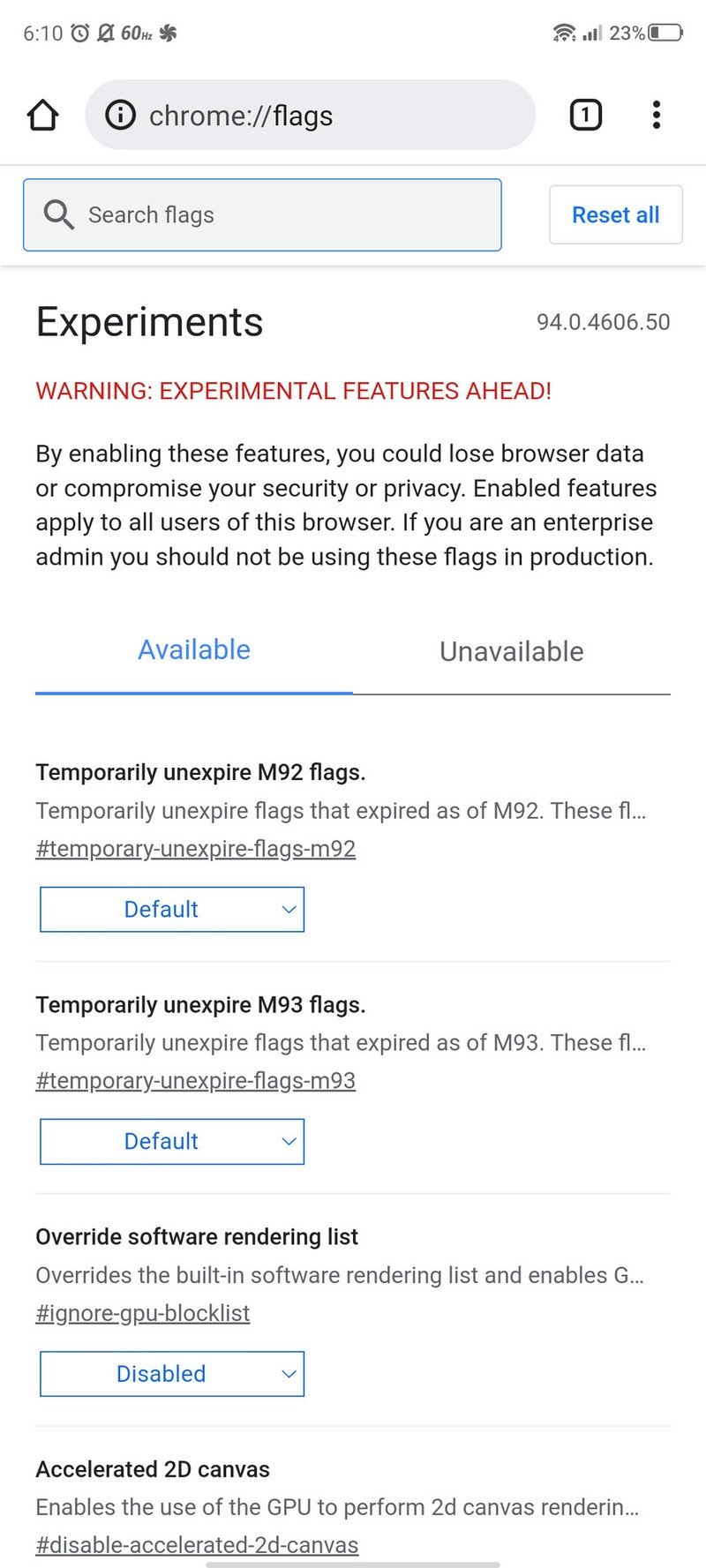This is a detailed screenshot from a mobile phone with a white background. In the upper left corner, grey text displays the time as 6:10 AM next to an alarm clock icon. Below it, "60W" is indicated, which might refer to wind speed. The upper right corner shows full Wi-Fi connectivity, a mobile signal strength of 3 out of 4 bars, and a battery level of 23%.

The main content of the screenshot highlights the 'Chrome Settings' page. At the top, the URL "chrome://flags" is displayed. Directly below, a grey search field reads "Search flags" accompanied by a small grey magnifying glass icon. To the right of the search field, a button labeled "Reset all" appears in blue font.

Further down, the text "Experiments" is shown in black font alongside the version number "94.0.4606.50." A warning in red font states, "Warning: Experimental features ahead." Below, black text cautions that enabling these features could result in lost browser data or compromised security and privacy. It also notes that these changes apply to all users of the browser and advises enterprise administrators against using these flags in a production environment.